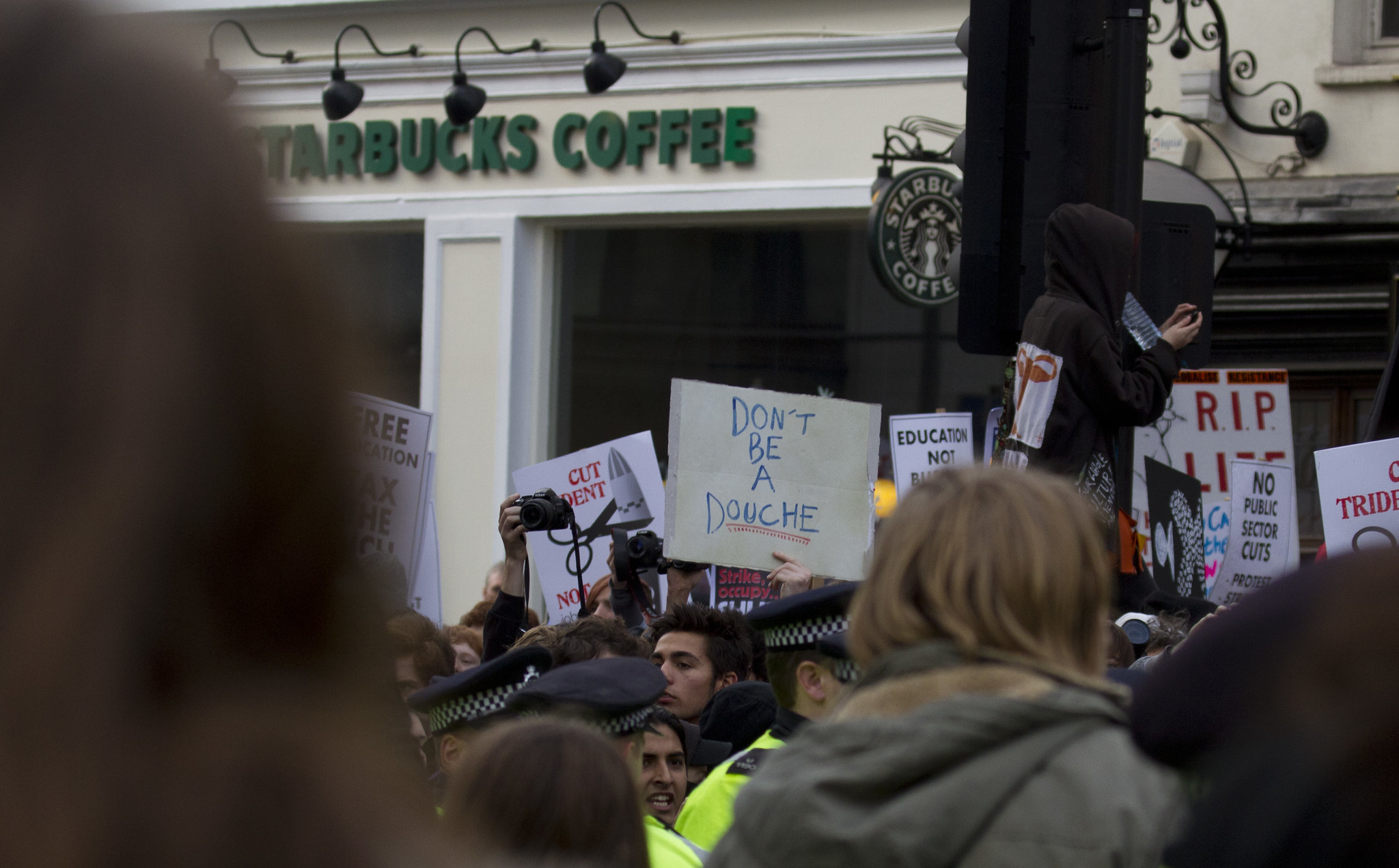The photograph captures a bustling urban protest taking place outside a Starbucks coffee shop during the daytime. The scene is filled with a chaotic jumble of people, some holding various protest signs while police officers in lime-yellow jackets and black hats navigate through the crowd. A blurred image of the backside of a woman with long brown hair partially obscures the far left of the frame. The Starbucks logo in green print is visible against the cream-colored storefront with four elongated lamps. 

Among the signs, one reads "Don't Be a Douche" in bold blue lettering with a red underline. Another sign states "Education Not," though the rest of the message is obscured by a woman's head. Other signs include "RIP Life" and "No Public Sector Cuts." One protestor appears elevated, either sitting or standing on a ladder, near a sign marked "RIP," seemingly touching a streetlight. Another individual is seen holding up a camera, capturing the scene over the heads of the crowd. The overall atmosphere is one of passionate dissent and disorder, centered around social and political issues.